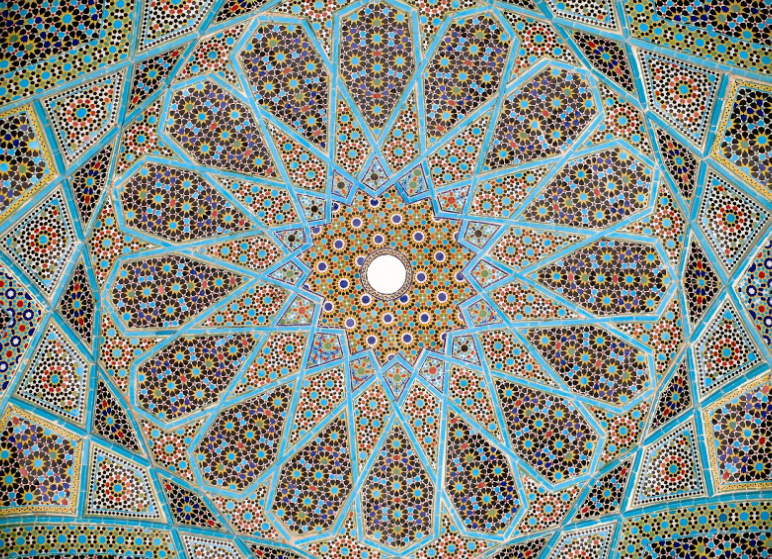This image features an intricate and vibrant kaleidoscope pattern, reminiscent of a colorful mosaic tile. Central to the composition is a star-shaped formation outlined in light blue, with a blank circle at its core. Surrounding this are layered stars filled with complex and colorful kaleidoscope designs that include tiny circles in shades of green and blue. The image includes a blue intersecting line motif, resembling a spirograph, threading through the design. Within the bustling arrangement, smaller brown and black tiles create a rich tapestry, accented by florets arranged in a diamond pattern that slightly tilts off-center. The overall effect is a mesmerizing blend of geometric precision and natural beauty, evoking the intricate artistry of Persian or Middle Eastern mosaics, albeit with a hint of digital abstraction.